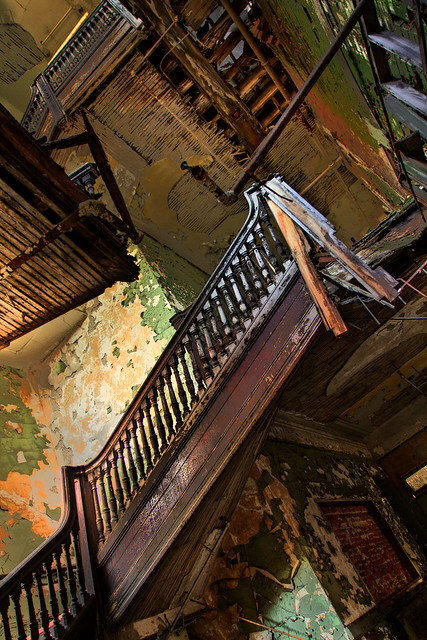This detailed image captures the interior of a dilapidated, abandoned house, highlighting its severely damaged and aged state. The main focus is on an old, wooden staircase with broken railings and missing steps, displaying deep chestnut hues beneath patches of peeling paint. The staircase, extending through two floors, reveals another set of stairs at the top of the image, partially obscured but similarly deteriorated. The surrounding walls, coated in chipped green paint interspersed with peeling layers revealing yellow and white beneath, add to the sense of decay. Exposed piping and hanging wood pieces further emphasize the long-standing neglect. The photo, taken at an angle, offers glimpses through the ceiling, showing wooden boards and supports that hint at a once-sturdy structure now succumbing to time.